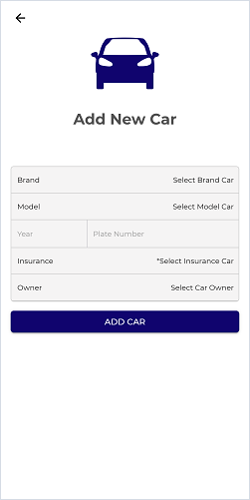The image features a white box bordered with a light blue frame. At the top of the box, there is a black arrow pointing to the left. Directly beneath the arrow is a dark blue icon of a car. Below the car icon, in black text, is the label "Add New Car."

The section below contains a series of light gray input boxes. The first input box is labeled "Brand" on the left side, with a placeholder on the right that says "Select Brand Car." Directly below, another input box labeled "Model" appears on the left, with "Select Model Car" as its placeholder on the right.

Continuing downward, the following row includes two more input boxes: "Year" on the left and "Plate Number" on the right. Below these, another row features "Insurance" on the left, accompanied by an asterisk, and "Select Insurance Car" as the placeholder text on the right.

Finally, the last row of input boxes includes "Owner" on the left and "Select Car Owner" as the placeholder on the right. Below all these input fields, there is a noticeable gap of white space.

At the bottom of the white box, there is a dark rectangular button with rounded edges. In the center of this button, "ADD CAR" is written in capital white letters.